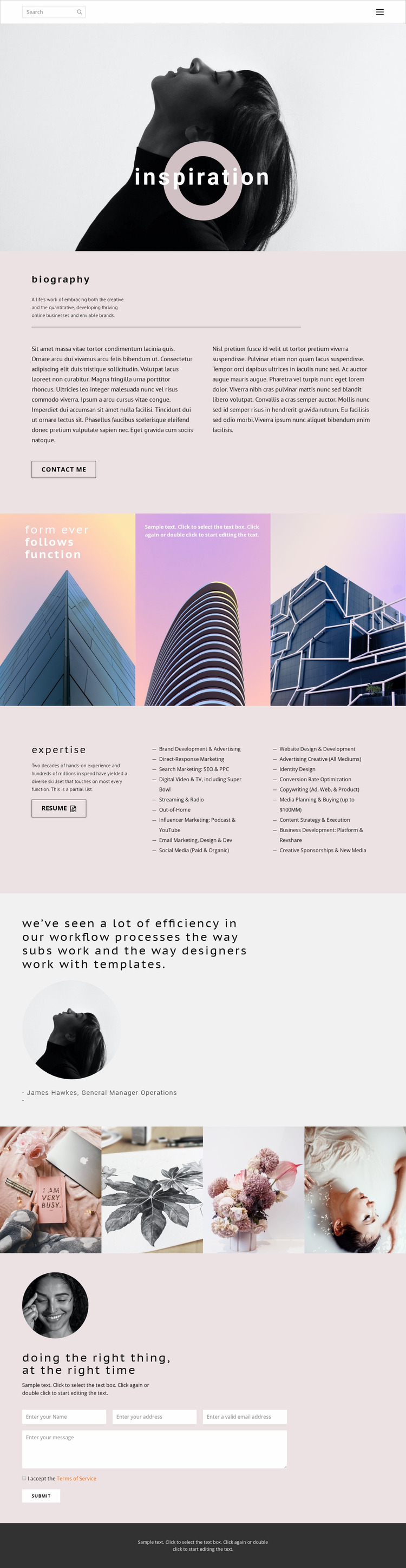The poster is a tall, vertically oriented design dominated by a theme of inspiration and productivity, set against a light beige or pastel-colored background. At the very top is a black-and-white image of a woman tilting her head back, gazing skyward with a white circle overlaid along with the word "inspiration." Below this is a biography detailing her journey, emphasizing her blend of creativity and quantitative skills in building successful online businesses and admired brands. The biography is flanked by two columns of text in very small font, which includes English phrases and what appears to be Latin placeholder text.

Following this, the poster is segmented into seven sections. The next section features three architectural images, each with their own pastel-colored backgrounds and accompanying text. The first image shows a skyscraper viewed from below against a sunrise gradient of yellow to orange, symbolizing growth and aspiration. The second image depicts an oval-shaped building with a purple-pink gradient background, while the third shows a black structure with white piping on a lavender backdrop.

Below the architectural images, another section labeled "Expertise" outlines the woman's extensive skill set from brand development and direct response marketing to search marketing and media planning, showcasing her comprehensive experience. This section directs viewers to a resume link and illustrates her prolific capabilities with specific areas of expertise listed.

Further down, there is another black-and-white image of the woman, once again looking upwards, next to four sentences of text that emphasize her achievements and philosophy. The final section is visually impactful, featuring four smaller images of flowers and artistic elements, with a circle image of the woman smiling underneath. This part of the poster continues the theme of "doing the right thing at the right time," and includes a user input section for name, address, email, and messages, alongside links to Terms of Service and a submit button, reinforcing the interactive and modern design of the poster.